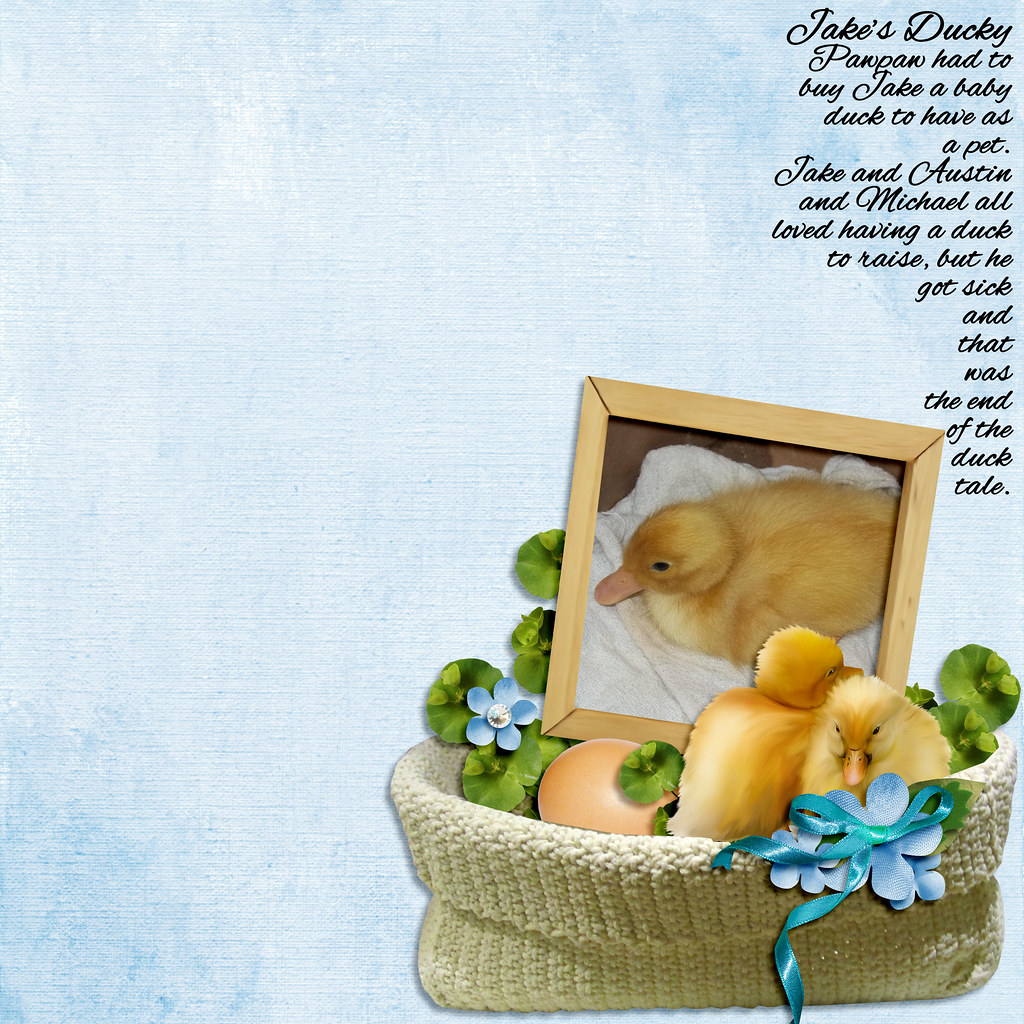The image features a softly textured, pale blue canvas background. In the bottom right sits a cream-colored, knitted basket adorned with blue flowers and a blue ribbon. Inside the basket are several fluffy yellow baby chicks and a small brown egg positioned to the left. The basket also contains some green leaves and clover. To the right of the basket, a framed photograph of a baby duck with pale yellow fuzz is nestled among the decorations. The wooden frame is accented by the same blue ribbon. In black cursive at the top right corner of the image, text reads: "Jake's Ducky. Pan Pan had to buy Jake a baby duck to have as a pet. Jake, Austin, and Michael all loved having a duck to raise, but he got sick and that was the end of the duck tale."